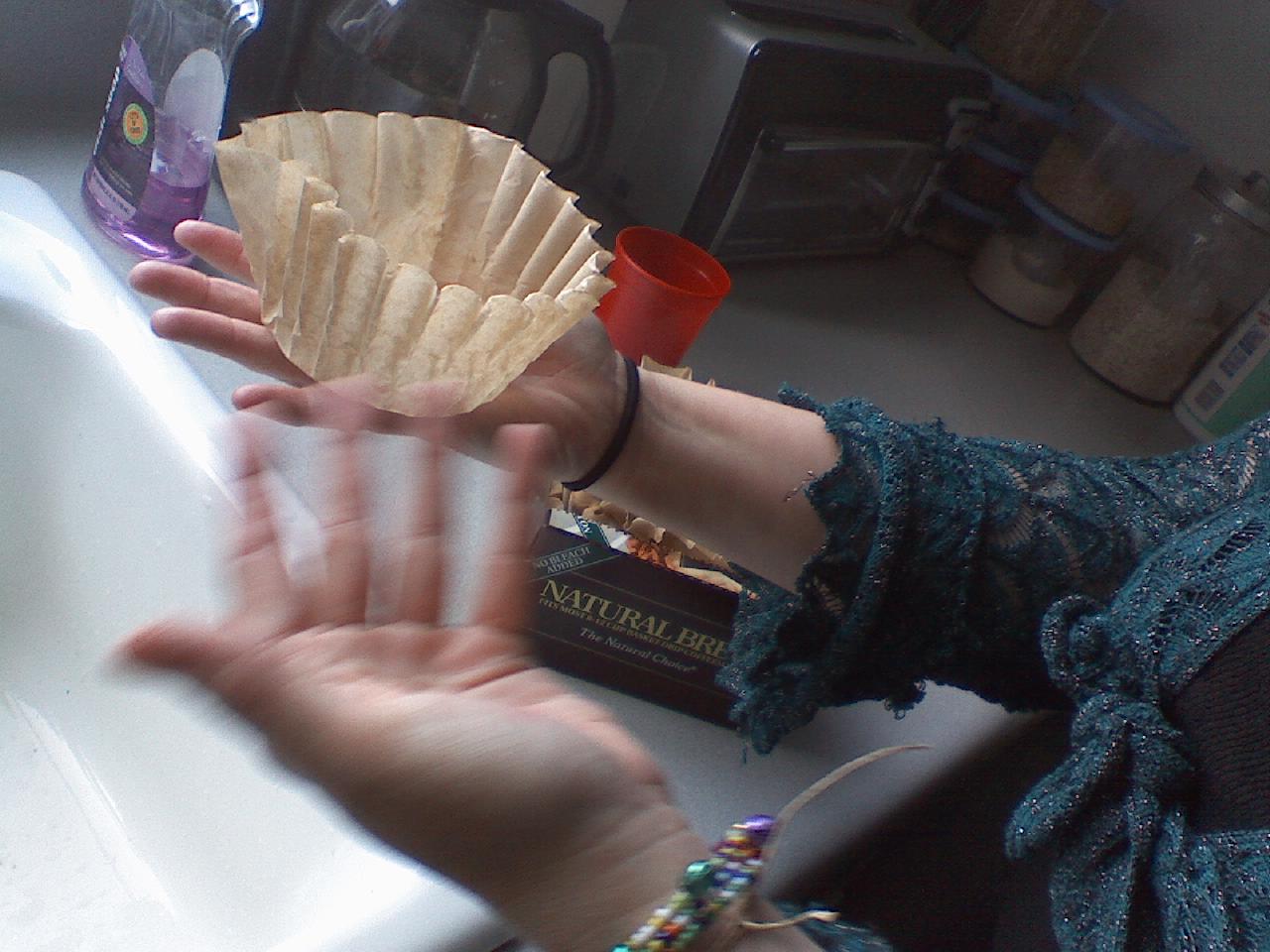In this detailed, motion-blurred photograph, a person stands at a kitchen counter, holding a used, tan coffee filter with their right hand. Their left hand is captured in mid-motion, appearing blurred, and is adorned with a multicolored beaded bracelet. They are dressed in a stylish green shirt, which features an elegantly designed soft and fuzzy fabric interwoven with mesh material, possibly with bits of glitter or sparkle. The shirt's sleeves are slightly rolled up to the middle of the forearms. A black hair tie is wrapped around their right wrist. The person is positioned in front of a gray kitchen countertop, with a white porcelain sink visible to the left. On the counter, there is a clear plastic bottle of pink dish soap, a seemingly used coffee pot, a silver toaster oven, and several spice bowls against the back wall. Additionally, a black box labeled with the word "natural" and a red cup are also visible on the countertop, contributing to the kitchen's bustling, yet homely atmosphere.